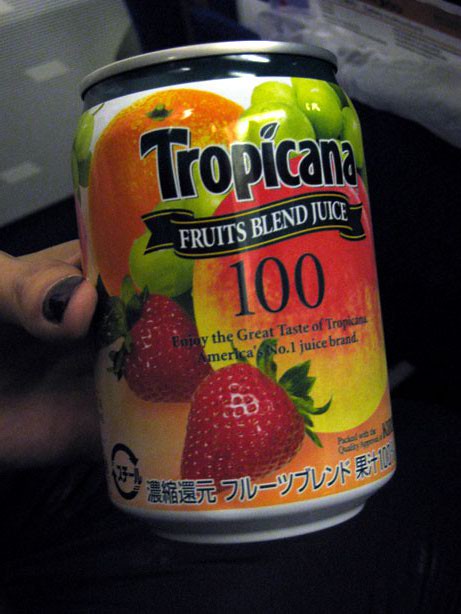In this image, a hand with black nail polish is holding a colorful can of 'Tropicana' beverage. The can features 'Tropicana' written prominently in black text. Below this, there is a black ribbon banner with the phrase 'Fruits Blend Juice' in white text. Underneath the banner, the number '100' is displayed in black text, followed by a smaller text that reads, 'Enjoy the great taste of Tropicana, America's number one juice brand'. Along the bottom of the can, there is an extensive amount of text in what appears to be an East Asian language, possibly Chinese, Japanese, or Korean. The can itself is adorned with vibrant images of various fruits, including oranges, grapes, pears, peaches, and strawberries, adding to its colorful and appealing design.